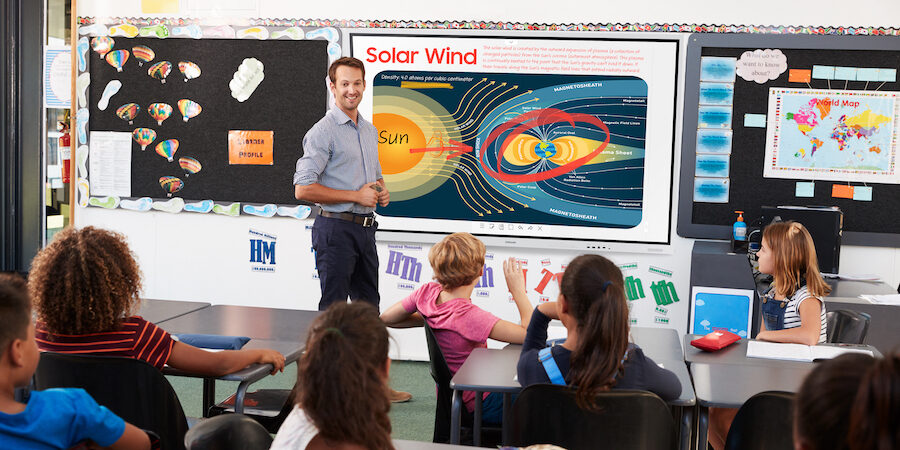In this detailed image of a grade school classroom, the diverse group of students, ranging in skin tone and dressed in colorful attire including red, pink, blue, and denim overalls, are seated attentively at their desks. At the front of the room stands the teacher, dressed in neatly pressed blue pants, a brown belt, and a light blue collared button-down shirt with the sleeves rolled above his elbows. He has short brown hair, a medium skin tone, and wears a welcoming smile as he instructs the class. Behind him are three distinct boards. The leftmost board is decorated with hot air balloons, clouds, and footprints around the border. In the center is a prominent poster that reads "Solar Wind," illustrating how the Sun's solar wind affects the Earth’s weather patterns with arrows and images. To the right, another board displays a world map along with a thought bubble and numerous sticky notes. The classroom scene captures a moment of engaged learning as the teacher explains the scientific connection between the Sun and the Earth's atmospheric conditions.